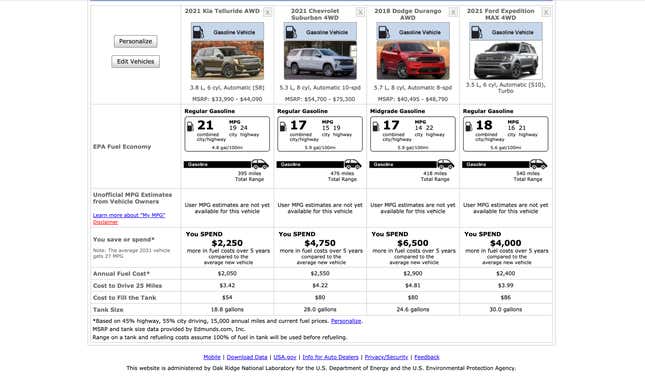This image depicts a dated-looking automobile comparison website or application, reminiscent of early 2000s web design. The interface consists of a simple HTML table on a white background with very light gray dividing lines, comparing four different SUVs. The table includes columns for various car specifications and costs, prominently focusing on fuel economy metrics such as EPA fuel economy ratings (listed as 18 mpg, 17 mpg, 17 mpg, and 21 mpg). 

At the top left corner, there is a section labeled "Personalize and Edit Vehicles," featuring clickable buttons that have a Windows 7 style appearance. The data includes other details like vehicle prices ($2,250, $4,750, $6,500, and $4,000), annual fuel cost, cost to drive 25 miles, cost to fill the tank, and tank size, emphasizing the importance of fuel efficiency and associated costs.

The image quality is low resolution and heavily artifacted, making it difficult to read some details, especially the blue hyperlinks at the bottom of the page. These hyperlinks are likely navigating options or additional resources related to the car comparisons. Despite the artifacting, the table's layout clearly aims to present an easy-to-read, side-by-side comparison of various fuel economy statistics and expenses for the displayed SUVs.